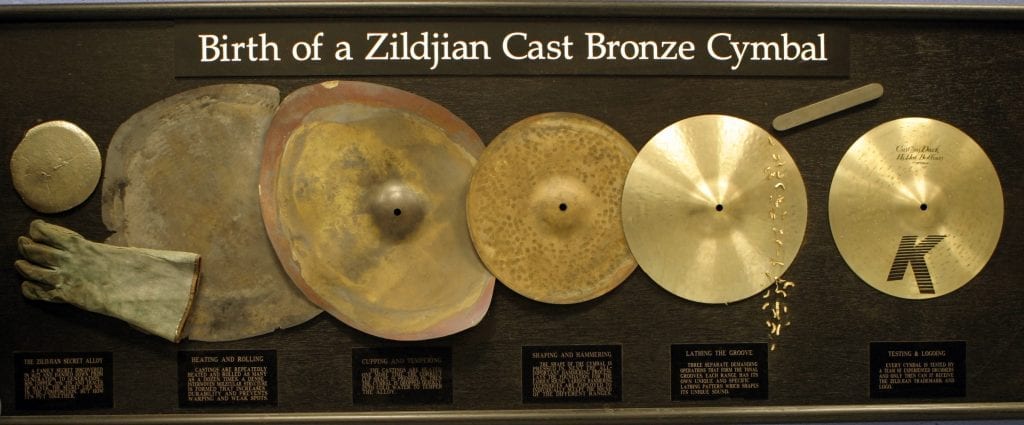This image showcases the captivating evolution of cymbals, illustrating their journey from ancient, rudimentarily shaped instruments to the refined modern versions. Titled "Birth of a Zildjian Cast Bronze Cymbal" at the top in white text, the photo captures six distinct cymbals arranged from left to right, highlighting their progressive development over time. Each cymbal is mounted with an explanatory plaque beneath it, though the text is illegible, it likely describes their era, composition, and manufacturing details. The first cymbal on the far left appears crude and irregularly shaped, accompanied by a pair of gloves presumably used in its creation. As you move towards the right, the cymbals become increasingly round, shiny, and polished, reflecting advances in craftsmanship. The final cymbal on the far right, adorned with a distinctive 'K' in black, epitomizes the sleek, modern design. The entire display is set against a dark brown background, and a tool can be seen at the top right, perhaps used in the cymbal-making process. This detailed exhibit, possibly part of an art collection, meticulously documents the transformation and refinement of cymbal design, demonstrating the significant strides in their development over the years.